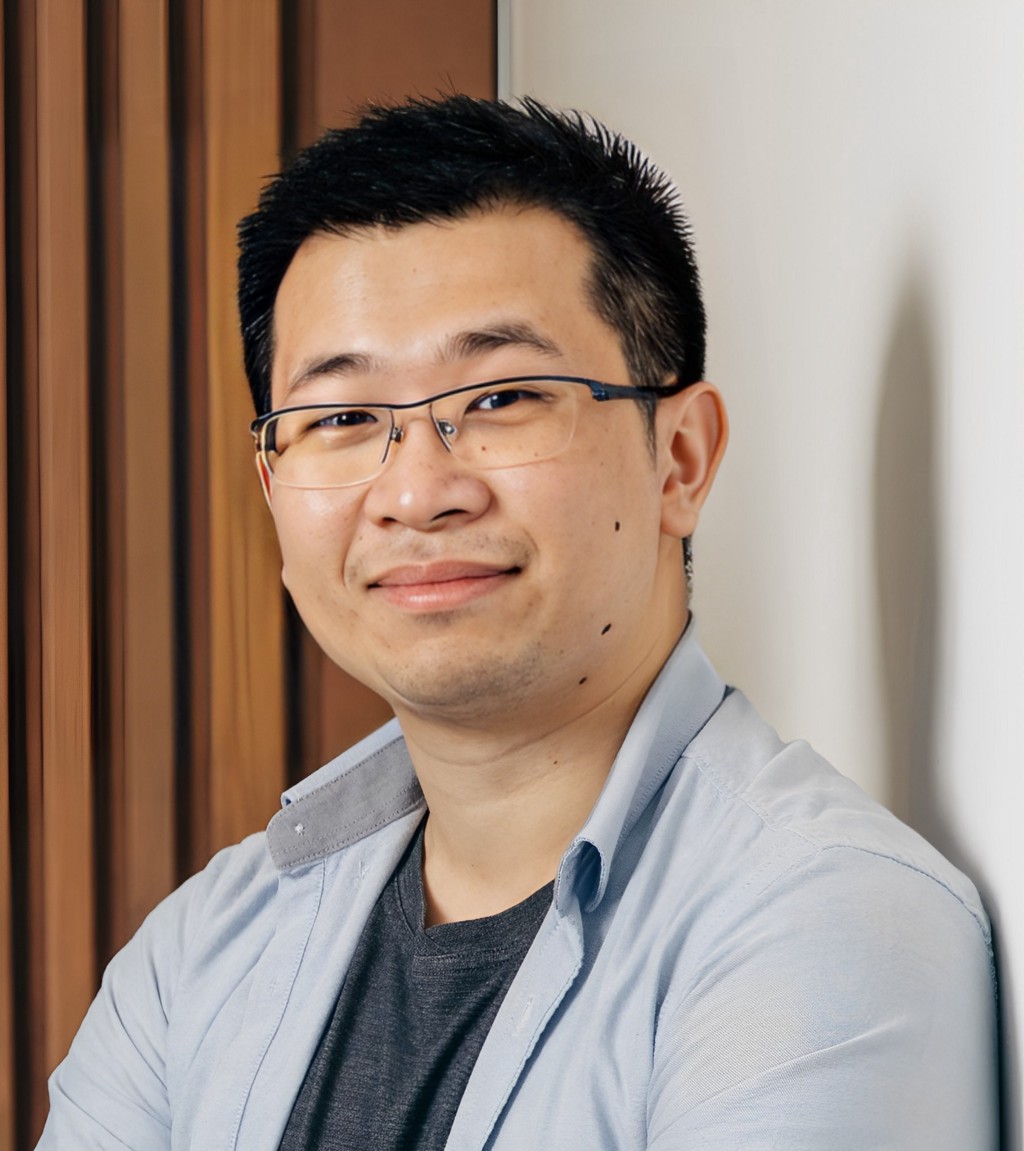This is a close-up photograph of a young man of Asian descent, likely in his mid-20s. He has dark, almost black, short cropped hair styled spiked up on top and clean-shaven face. The man has dark black eyebrows and three prominent moles aligned vertically on the left side of his face. He is wearing narrow-rimmed, wire-framed glasses that sit slightly low on his nose. The man is smiling and appears relaxed. His outfit consists of a gray round neck t-shirt layered beneath a light blue, long-sleeved, button-down collared shirt worn open. The photograph captures him from the chest up, with his body facing slightly left but his head turned towards the camera. The background is split into two different textures; the right side is a plain white wall, casting a faint shadow of his silhouette, while the left side features vertical wooden panels that resemble wood beams. The juncture of the white wall and the wood paneling aligns directly behind the young man's head, providing a distinct backdrop that contrasts yet complements his appearance.